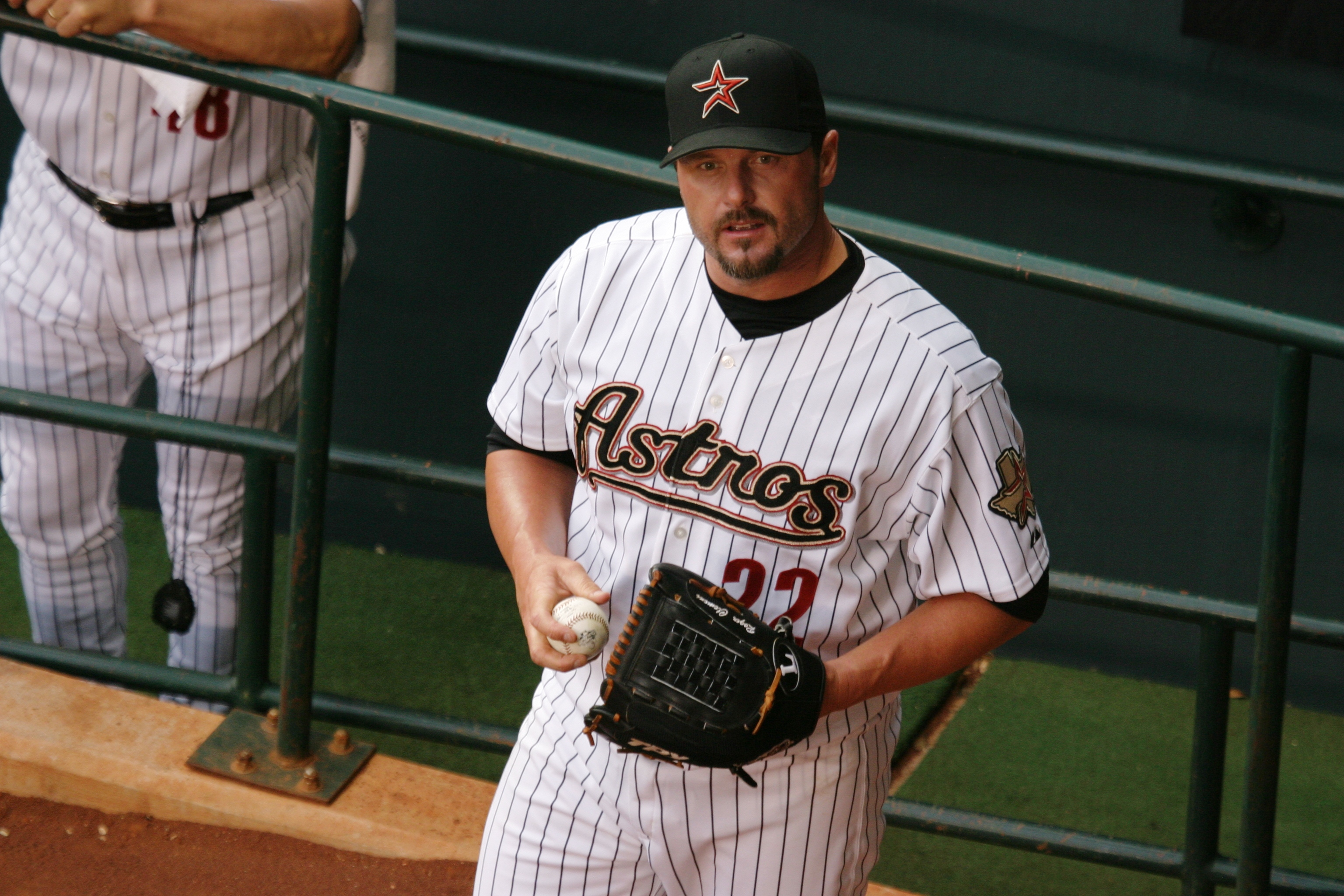The image is a detailed photograph capturing baseball pitcher Roger Clemens during his tenure with the Houston Astros. Clemens, identifiable by his distinctive brown goatee, is depicted standing near a green metal railing in what appears to be the bullpen of a stadium. He is adorned in a full Astros uniform: a white jersey with black vertical pinstripes, the word "Astros" emblazoned across the chest in bold black letters with a red outline, and the number 22 in red. The jersey also features a patch in the shape of Texas on the left side. Clemens is wearing a black cap with a red star logo. He is gripping a baseball in his right hand and has a black pitcher's mitt on his left. Behind him, another player in a similar uniform is partially visible. The background includes a mix of green turf and dirt, highlighting the bullpen setting.